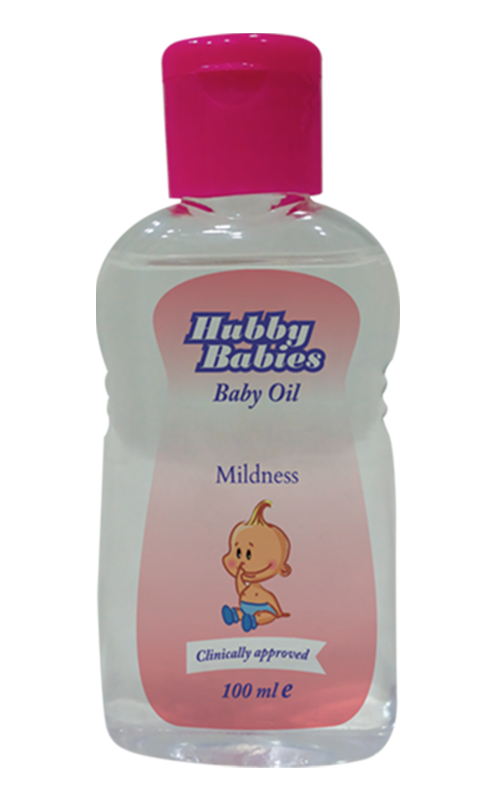In this image, a bottle of Hubby Baby's Baby Oil is placed against a completely white background, and the object occupies the majority of the frame with a zoomed-in view allowing for detailed examination. The clear bottle, filled to the top with liquid baby oil, is in pristine condition, suggesting it is brand new. The cap atop the bottle is pink and securely closed. The label features a combination of colors including blue, white, and pink. Prominent text on the bottle reads "Hubby Baby's Baby Oil," "Mildness," and "Clinically Approved" in blue and white letters. A small, white banner at the bottom of the label shows "100 milliliters" in blue text. Additionally, there's a picture of a cute baby with a lock of hair, wearing a diaper and booties, possibly sucking a thumb, set against the clear background of the bottle. The baby’s skin tone is light brown. The image, with its clean presentation and high level of detail, resembles a product photograph suitable for a pharmacy website.